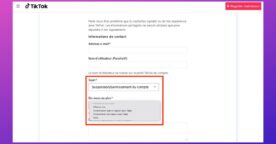This image is a small screenshot taken from a computer screen. The background gradually transitions from a pinkish hue at the top to a deeper purple towards the bottom. A prominent white rectangle is centered in the image, adorned with the word "Tic-tac" and a musical note icon in the upper corner.

Towards the right side of this white rectangle is a red rectangular button, though the text inside it is too blurry to decipher. Below the top section, a few sentences are visible, with some segments bolded in black for emphasis, situated around the middle of the image. Additional black text appears beneath these sentences in a smaller font. 

An orange-lined rectangle frames some content inside the white rectangle, including a search bar where a user has typed something. Finally, below this search bar, there are four lines of smaller black text.